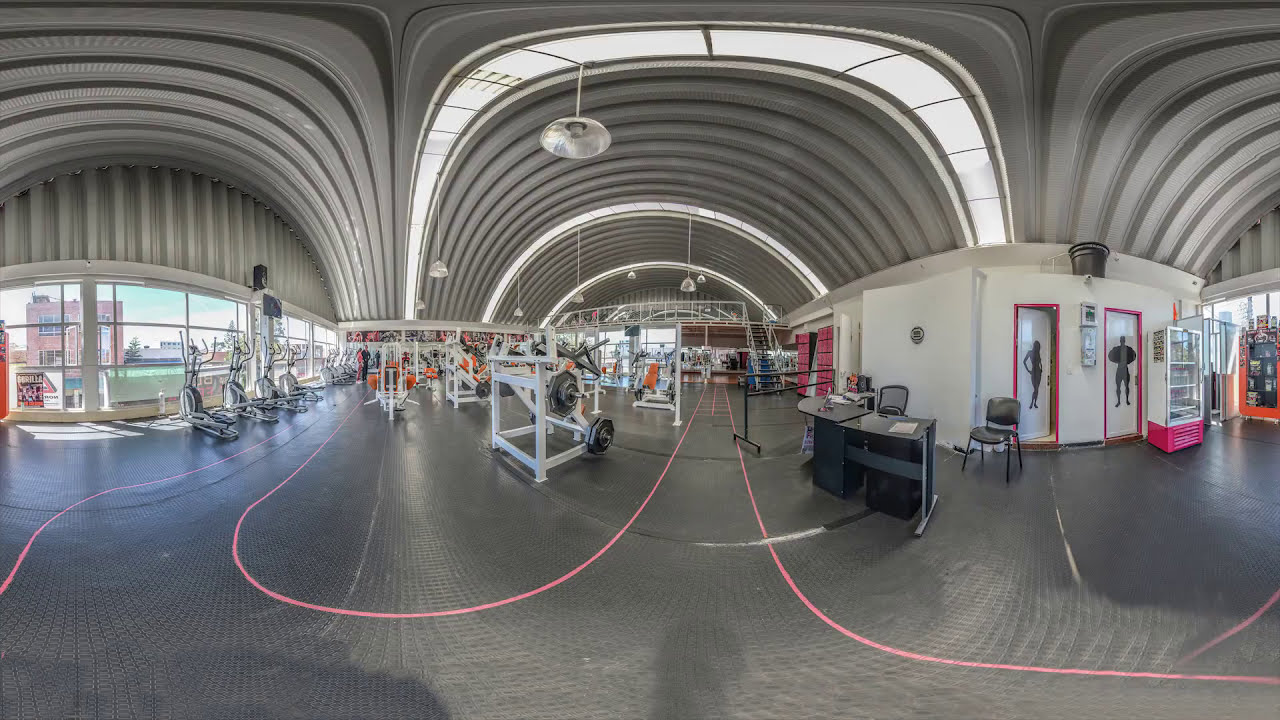The image showcases a spacious gym set in a modern, industrial environment with arching metallic grey ceilings and dark grey floors. Various gym equipment is scattered throughout, including ellipticals, treadmills, bench press stations, and weights housed in metal frames, featuring both circular and hexagonal plates. A distinct pink line is marked on the floor to guide pathways through the equipment.

To the right, there is a desk accompanied by two black chairs, indicative of a gym worker’s station. Behind the desk, two bathroom doors are visible – one with a silhouette of a woman and the other with a black outline of a man, partially open. Adjacent to these, vending machines are stationed, potentially offering refreshments and other fitness-related items.

The left side of the image features a large horizontal window spanning the building’s wall, flooding the gym with natural light and offering views of the outside cityscape. The sunlight reflects off the shiny black rubber flooring, adding warmth to the space. Several cross trainers with raised steps and handlebars are positioned near the window. A stairway at the center hints at a second level within the gym, enhancing the sense of depth in this 360-degree panoramic view that slightly distorts the overall perspective.